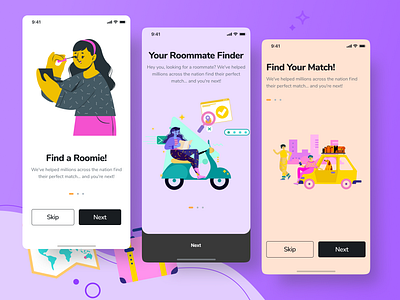The image is a small, square advertisement showcasing a roommate-finding app. It features three vertically aligned, phone-sized screenshots against a solid purple background. Each section is distinct:

1. The leftmost section has a white background and depicts an animated woman with dark hair, a grayish sweater, and pink pants. She appears to be using a phone, with the text "Find a Roomie" written above accompanied by skip and next buttons.

2. The middle section sports a light purple background with the header "Your Roommate Finder." It displays an animated girl in a blue shirt and black pants riding an aqua-colored scooter, along with a portfolio icon containing a magnifying glass and checkmark. This section also includes skip and next buttons at the bottom.

3. The rightmost section, set against a tan backdrop, is labeled "Find Your Match!" It portrays a computer-generated scene of a yellow car with luggage on top. A person, dressed in yellow, is standing beside it, and another individual is sitting on the car's hood with a dog inside. This scene also features the familiar skip and next buttons.

The purple background includes subtle elements like a single star, a briefcase, a world map, and a swirling design, enhancing the overall aesthetic.